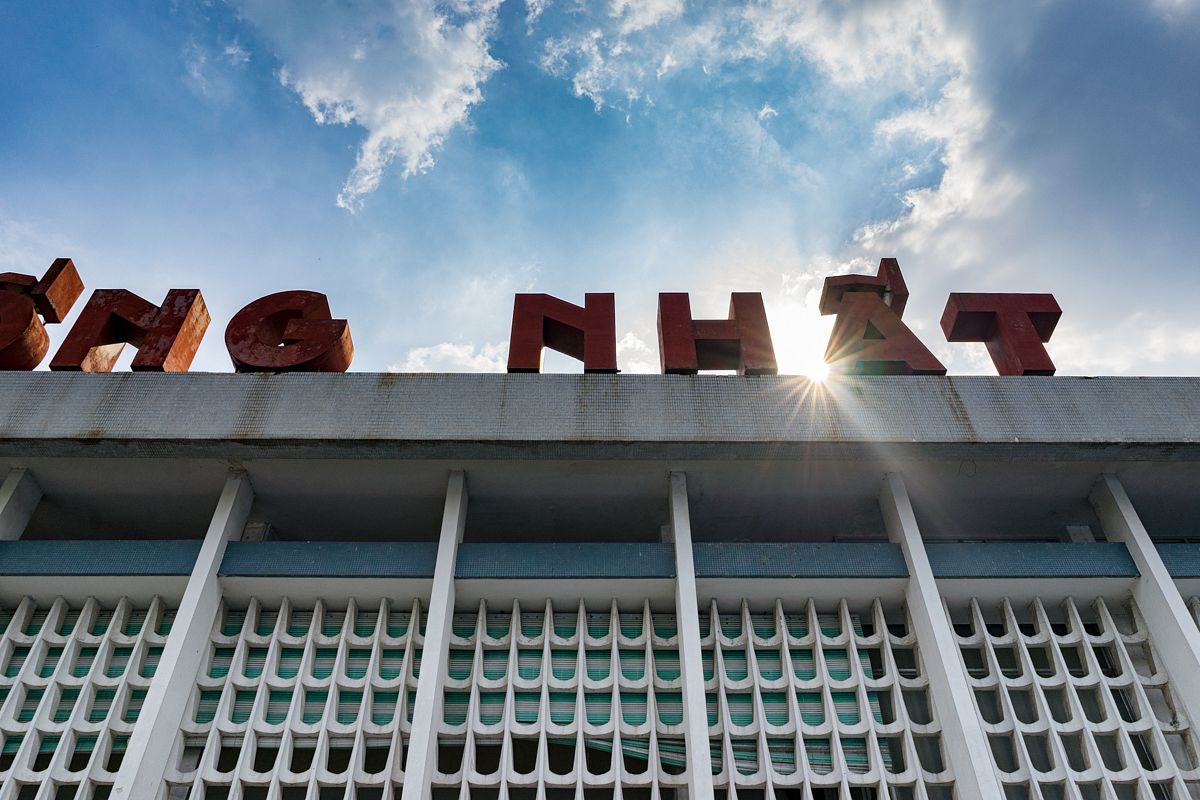This photograph captures a striking architectural scene set against a bright blue sky dotted with fluffy white clouds. The sunlight beams warmly, accentuating details of the structure. At the top, large red block letters dominate the view, with rays of sunlight streaming through the space between the "H" and "A." The roof's edge appears somewhat grimy, suggesting a lack of recent maintenance. Below this, a series of white columns support a bluish horizontal section, adding a decorative element to the facade. The lower part of the building features triangular peaks in a white framework, standing out against a backdrop of teal and white coloring. Overall, the building exudes a sense of faded grandeur, its red lettering showing signs of peeling, echoing the structure's evident state of disrepair.